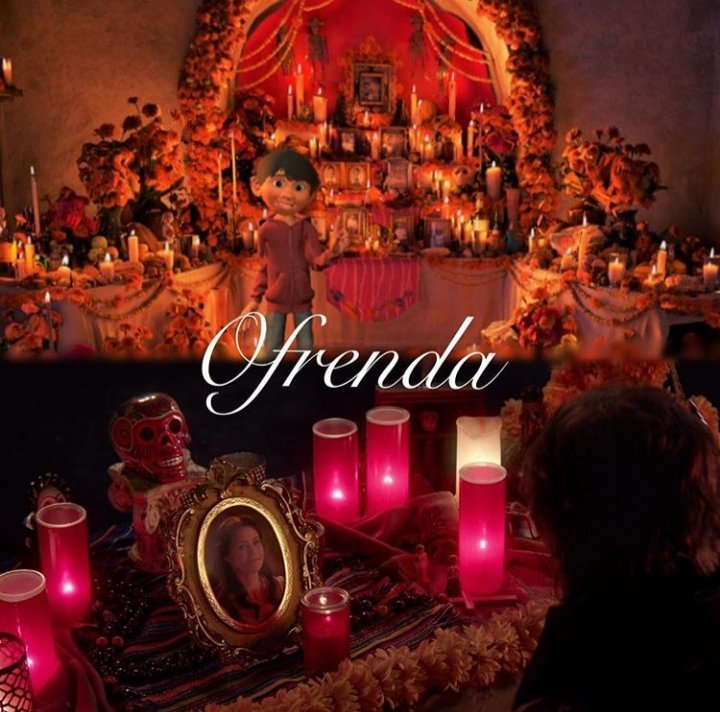The image depicts an elaborate and meticulously decorated altar, set against a dark backdrop. Shelves adorned with an abundance of candles of various shapes and sizes, vibrant flowers, and rich fabrics fill the scene. In front of these shelves, two tables loaded with similar decorative items proceed towards the foreground, where yet another table brims with glowing candles and floral arrangements. A round picture frame holding a photo of a woman is a focal point on the table. The background features an arch embellished with flowers, creating a grand setting for the arrangement. A small figure of a young boy with dark hair, wearing a red hoodie and gray pants, stands in front of the shelves, with the words "Oh Frenda" written across the image above him. Additionally, a glass skeleton head sits atop a box near the picture of the woman. More lit candles, draped in pink hues, add warmth and light to the scene, emphasizing the solemn and celebratory atmosphere of the altar which appears to serve as an ofrenda.